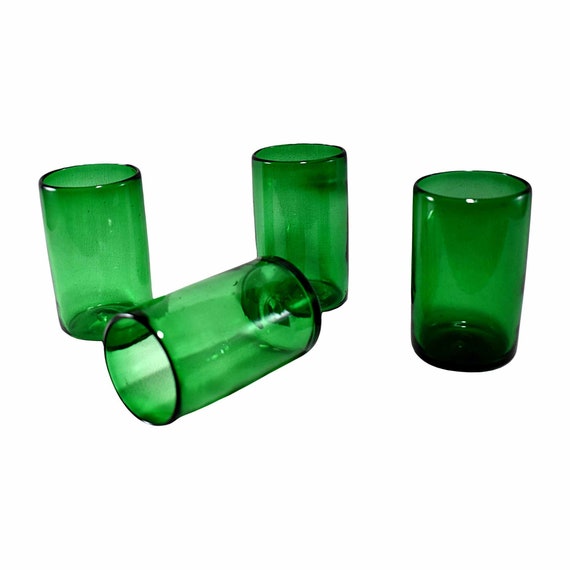The image displays four transparent green glass drinking glasses arranged against a plain white background. Three of these glasses are standing upright in a line: the first glass is on the left, the second glass is further back to the right of the first one, and the third glass is aligned with the first but positioned further forward. The fourth glass, slightly to the left of the center, lies on its side with its mouth pointing towards the southwest direction. All four glasses exhibit a deep, unique green color and are see-through, revealing that they are empty. These glasses, approximately eight inches tall and capable of holding around 16 ounces, seem robust, likely suitable for a bar setting. Subtle light reflections are visible around the rims, particularly on the glass that's on its side.